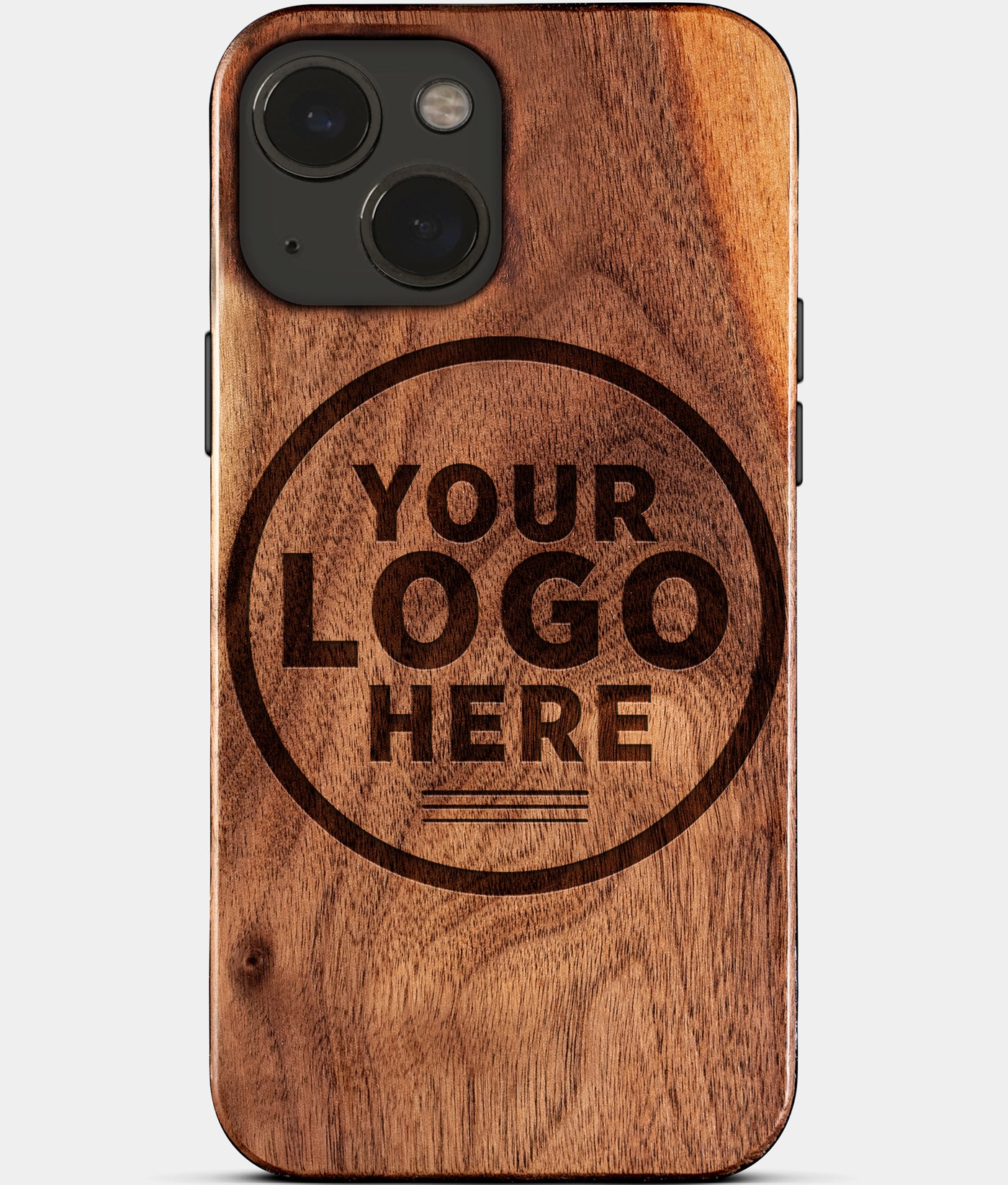This portrait-layout image showcases an iPhone with a wooden-like, dark brown cell phone cover set against a white background. The cover prominently features a darker circular area in the center with the text "Your Logo Here" in three lines. Below the text are three black lines. The iPhone’s dual cameras and flash are visible in the upper left corner, along with a single black button on the left side and two black buttons on the right. The text "Logo" in the center is the largest, emphasizing where a custom logo can be placed.